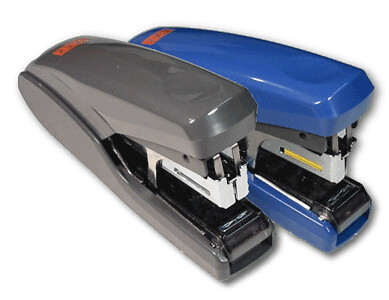The photograph showcases two small staplers, approximately four inches long, positioned on a plain white background. One stapler is gray, while the other is a medium blue. Both are of the same brand, likely Bosch, as indicated by the obscured orange logo on the back end of each stapler. The logo, although blurry, suggests a common design and model. The staplers exhibit a reflective silver upper section, where paper is clamped to staple, and a long black piece underneath. Both staplers appear open and ready for use. Of note, the blue stapler contains a visible cartridge of yellow staples. The arrangement gives the impression that the gray stapler may be slightly overlaid on the blue one, creating a somewhat incongruent but still organized display.